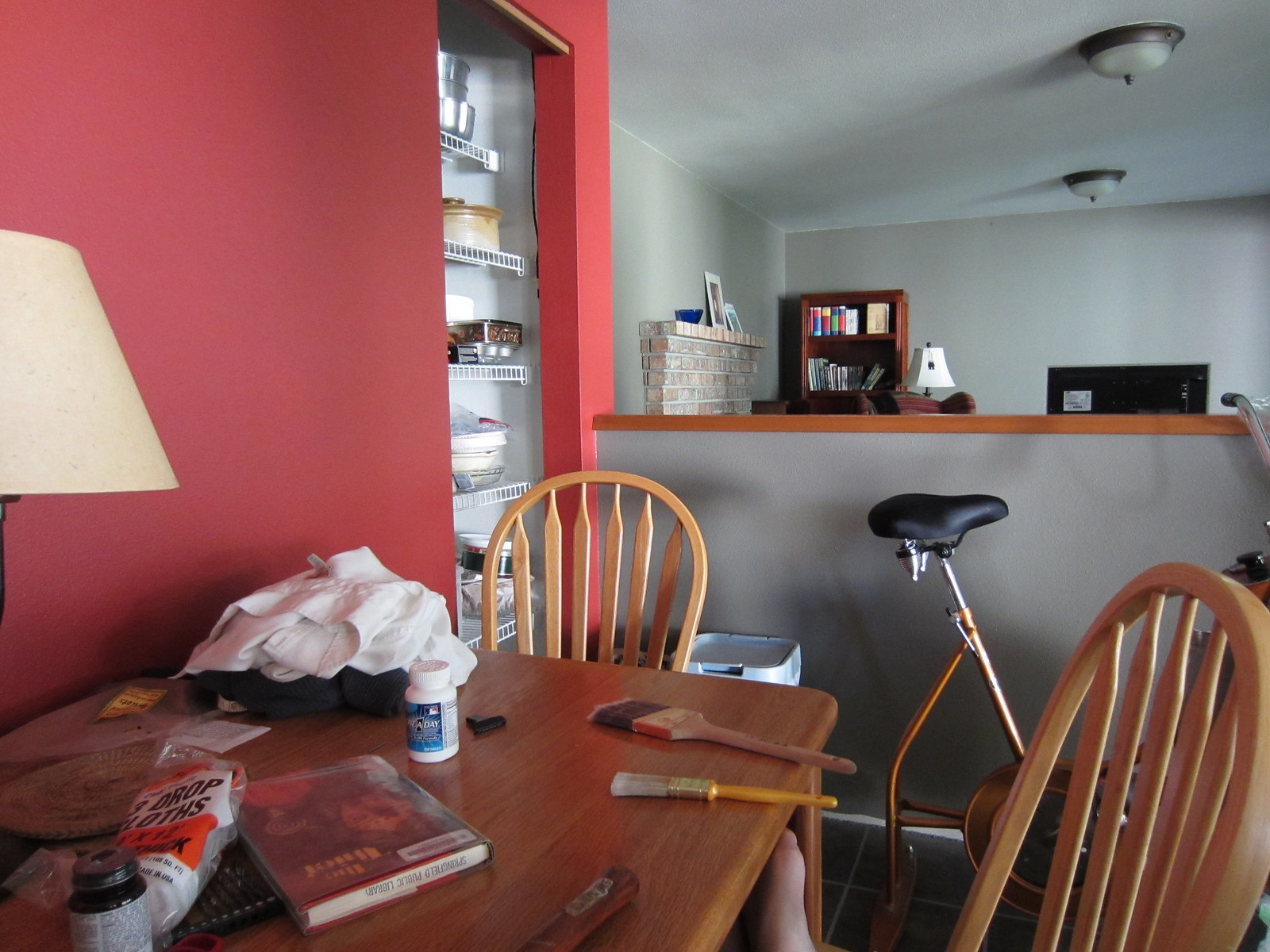This image captures a snapshot of a cozy dining room that opens into a living room, illustrating a layered blend of both spaces. 

In the far background, partially obscured by a central dividing wall, the top half of a wooden bookshelf stands out, anchoring the scene with a touch of rustic charm. On the bookshelf’s top shelf, a collection of colorful books adds a sprinkle of vibrancy, while the lower visible shelf holds a neat array of thinner volumes or records, hinting at the homeowner’s interests. 

Adjacent to the bookshelf on the left, the upper portion of a brick fireplace mantle comes into view, adorned with framed photographs that lend a personal touch to the space. To the right of the bookshelf, the tops of a lamp and a chair peek out, completing the glimpse into the cozy living room.

Moving to the foreground where the photographer is situated, the lower half of the scene is dominated by a wooden dining table with two chairs. The table is an eclectic workspace, scattered with folded clothes, paint brushes, a book, various tools, and an assortment of other items, reflecting an atmosphere of creativity and daily life.

Immediately in front of the dividing wall, a stationary bicycle adds a functional element to the room, its seat pointing towards the camera. To its left, the scene transitions into a more utilitarian corner with white plastic pantry shelves stocked with various pans, emphasizing the practical side of the home. The wall behind these shelves is painted a bold red, contrasting sharply with the gray hue of the fireplace wall, delineating the two distinct spaces within the home.

A lamp situated on the far left edge of the table brings additional warmth and illumination to the dining area, rounding out this intricately detailed depiction of a harmonious yet multifaceted living and dining space.